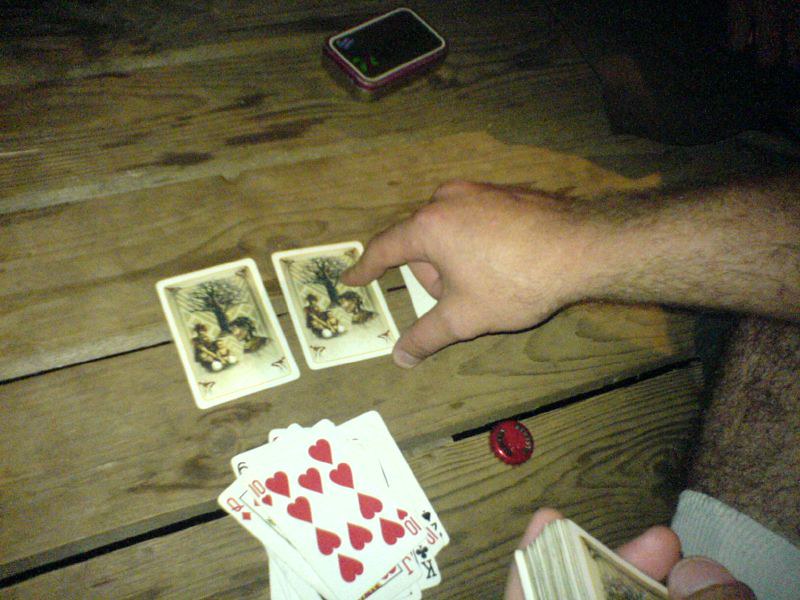A group of people are engaged in a game of cards on a wooden deck. In the foreground, a person with a hairy leg, suggestive of a man, sits with white socks partially visible. His hand, notably tanned and holding the deck of cards, extends into the frame. The deck's top card is the ten of hearts, followed by the queen of diamonds, and partially obscured behind them, a six, all arranged in a mixed sequence of red and black. Clearly visible is a joker, a king, and a two amidst the cards. The individual is in the process of placing two cards face down, revealing their intricately designed backs. Nearby, an open box or tin, presumably the original packaging for the cards, lies in the background. Additional details include a red bottle cap and noticeable stains on the brown wooden planks, adding texture and context to the scene.